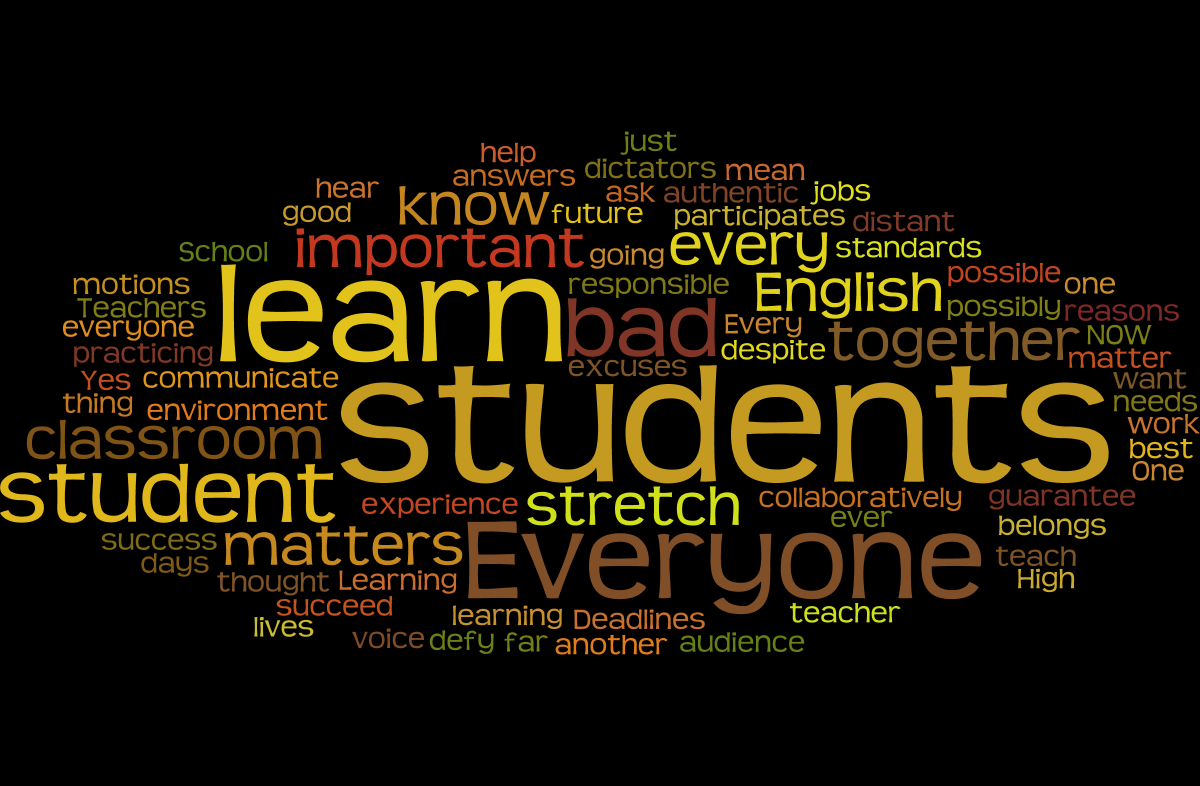The image features a word cloud on a stark black background, with varying text sizes and colors, from shades of yellow, orange, red, to browns, imparting an almost autumn-like feel. The dimensions are akin to a high-definition TV, wider than it is tall. Dominating the center are the largest and most prominent words "learn" and "students" in bold yellow hues. These central words are surrounded by an array of other related terms like "classroom," "communicate," "responsible," "English," "standards," "everyone," "bad," "excuses," and "succeed" among others, arranged in a loose oval shape. The words vary in size, indicating their relative importance or frequency, with "students," "learn," and "everyone" standing out noticeably. Smaller words like "help," "answers," "future," and "important" are scattered throughout, contributing to the educational theme, creating a layered and textured visual composed entirely of text elements related to learning and education.